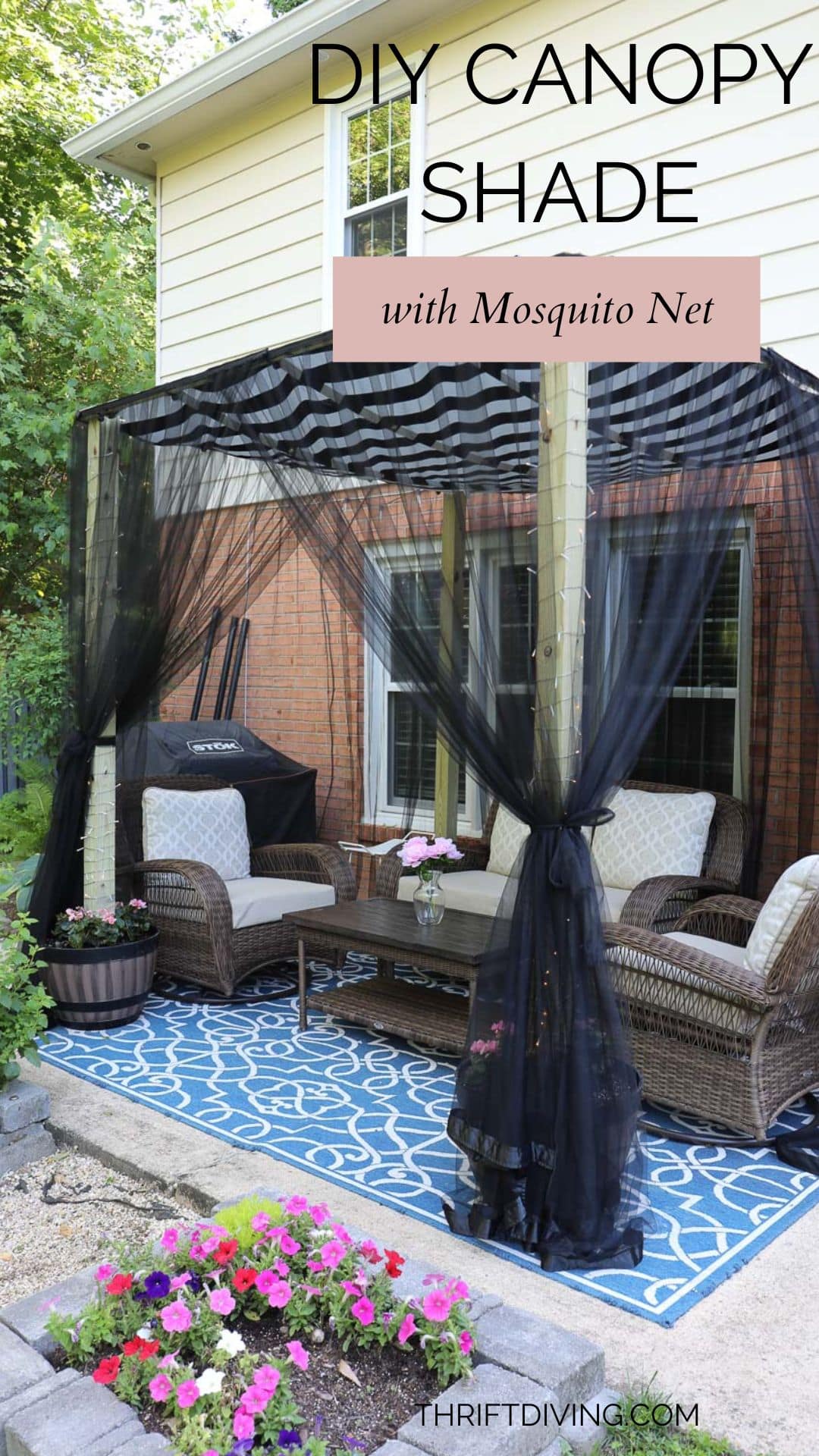In the advertisement image, a DIY canopy shade is prominently showcased with black, thin, large text. Below this, in a puce-colored rectangle, it reads "with mosquito net" in italics. The scene is set in the backyard of a standard suburban home, characterized by its upper beige paneling and lower red brick section, complete with white trim windows.

The backyard features an inviting arrangement of outdoor furniture, including a mix of wicker chairs and a small couch, complemented by a brown coffee table hosting a vase of pink flowers. This cozy setup is set atop a blue and white geometric-patterned rug. The canopy overhead, with its black lace mosquito netting, can be untied from the posts in each corner to enclose the entire area. Additionally, the canopy roof boasts a stylish black and white striped design.

A flower bed in the foreground blooms vibrantly with various pink, red, blue, yellow, white, and purple flowers, enhancing the serene and picturesque quality of the suburban backyard.